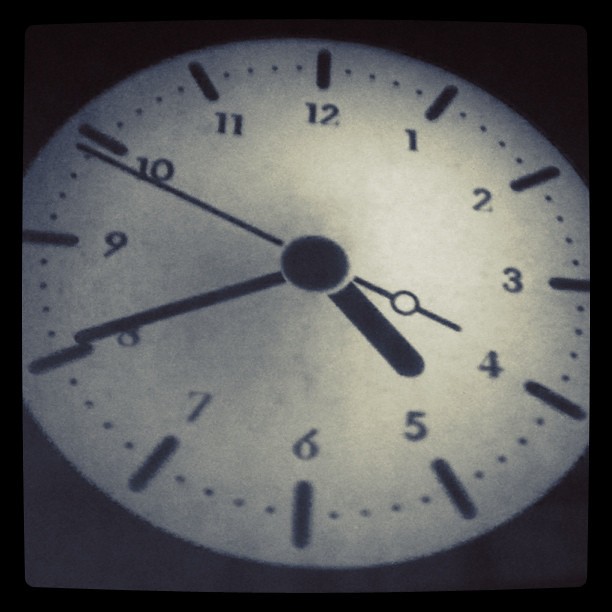In this striking black and white photograph, the focus centers on an illuminated clock face, suggesting it might be part of a larger clock tower structure. The round clock face, glowing against a deep black backdrop, draws immediate attention. All its components—the numbers, hour and minute hands, and minute markers—are rendered in bold black, creating a sharp contrast against the luminous white background of the clock face itself. A light source, placed just between the 12 and 3 o'clock positions, further highlights specific details. The image is closely cropped, with only portions of the 9 and 3 o'clock numerals visible, hinting at the partial extension of these details beyond the field of view. Framing the composition is a substantial black border, adding to the photograph's classic and dramatic ambiance.